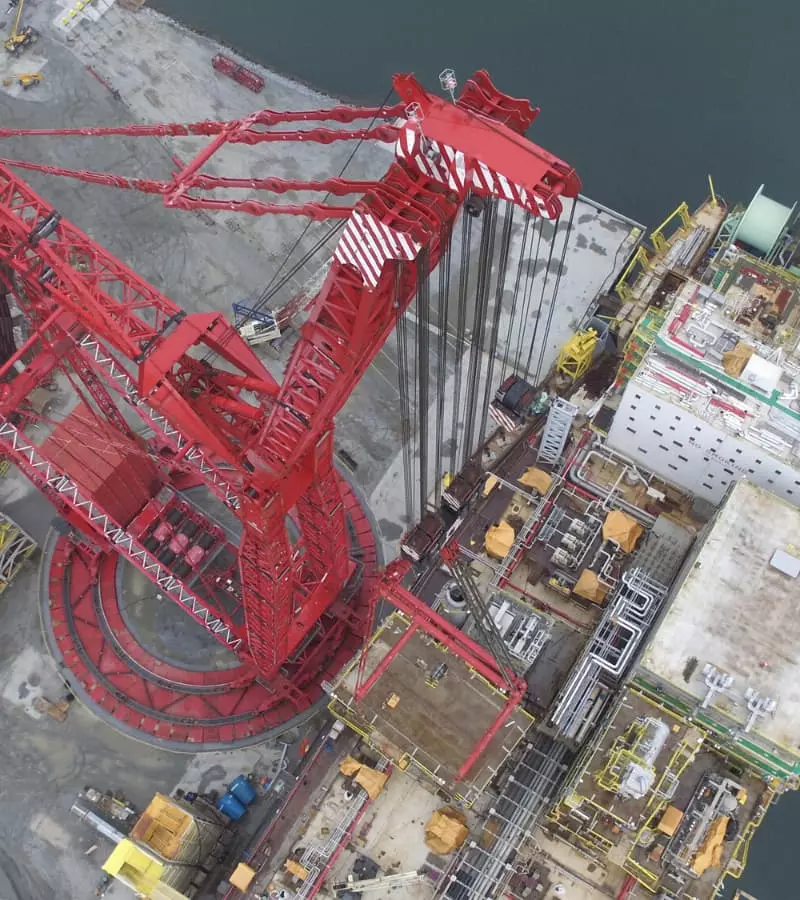This aerial photograph captures a bustling industrial waterfront site dominated by a gigantic red crane equipped with black-lined cables and a platform. The crane, a permanent fixture on the dock, is likely used for loading or unloading shipping containers, though no containers or ships are visibly present. Surrounding the crane, there are multiple white buildings, parking lots, and extensive yellow-piped infrastructure sprawling across a large concrete area. Small barrels can be seen underneath the crane, enhancing the sense of industrial activity. The image also features visible water bodies at the top and bottom right-hand corners, confirming the site's proximity to a large body of water, potentially an ocean or lake, though no boats are visible.